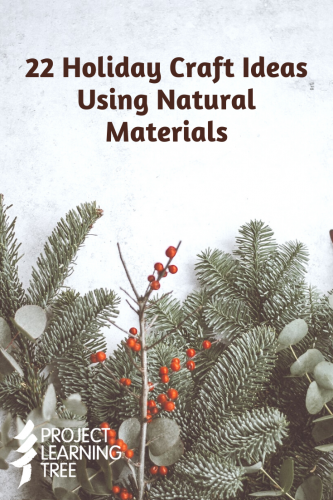This detailed poster design focuses on promoting "22 Holiday Craft Ideas Using Natural Materials." The central visual element is a hand-drawn or artistically depicted scene featuring lush evergreen branches adorned with vibrant, round red berries. The background is a clean, white canvas that allows the natural greenery and striking berries to stand out. The main title at the top of the poster is boldly displayed, announcing "22 Holiday Craft Ideas Using Natural Materials" in a brown font. At the bottom left corner, in all capital white letters, it states "PROJECT LEARNING TREE," accompanied by a logo that represents Project Learning Tree. The whole composition maintains a harmonious natural aesthetic, with the evergreen branches and the striking red berries creating a festive and organic visual appeal.